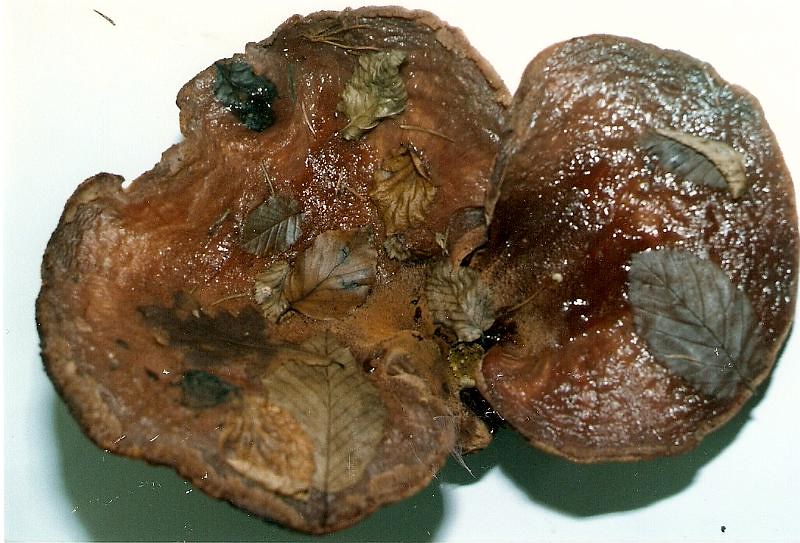The image depicts a meat-like object, possibly resembling an open clam or a rock slice, positioned on a white surface, likely a plate. The object appears dark brown and glistening with a glossy, almost oily texture, suggesting it is very moist. Embedded within or scattered on top of this object are decomposing, burnt leaves in varying shades of grey, green, and pale yellow. These leaves add a sense of decay, and their presence indicates they have darkened and decayed over time. This meat-like structure has a slightly gooey or gel-like interior, especially noticeable towards its darker, hinged end, where the substance appears to have oozed. The overall composition includes shadows beneath the object, further distinguishing the glazy, detailed texture of the food against the clean, white background.